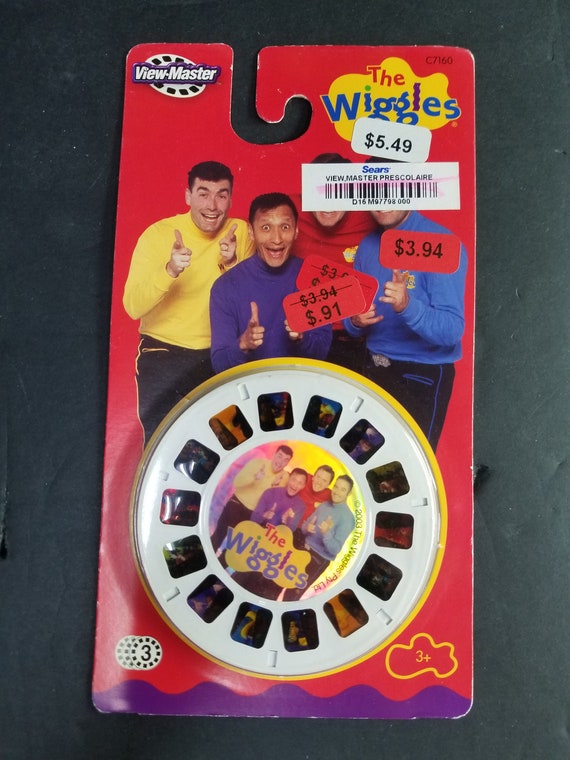The image shows a vintage Viewmaster slide package featuring The Wiggles, displayed against a dark grey, possibly black, background. The top left corner of the package prominently features the Viewmaster logo, while the top right showcases The Wiggles' logo in their distinctive playful font within a yellow blobby shape. Below the logos is the highlight of the package: a shrink-wrapped round Viewmaster slide reel with several miniature photos around its perimeter and a central image of The Wiggles—four smiling men dressed in yellow, purple, red, and blue shirts. Above this, The Wiggles give a thumbs-up, adding to the cheerful aesthetic of the package. Various price tags are visible on the packaging: an initial $5.49, then marked down to $3.94, and finally reduced to $0.91, revealing the progressive discounting over time. A smaller tag denotes it as suitable for ages 3 and above. This nostalgic toy item is complete with a barcode and is still preserved in its original packaging, hinting at its collectible value.